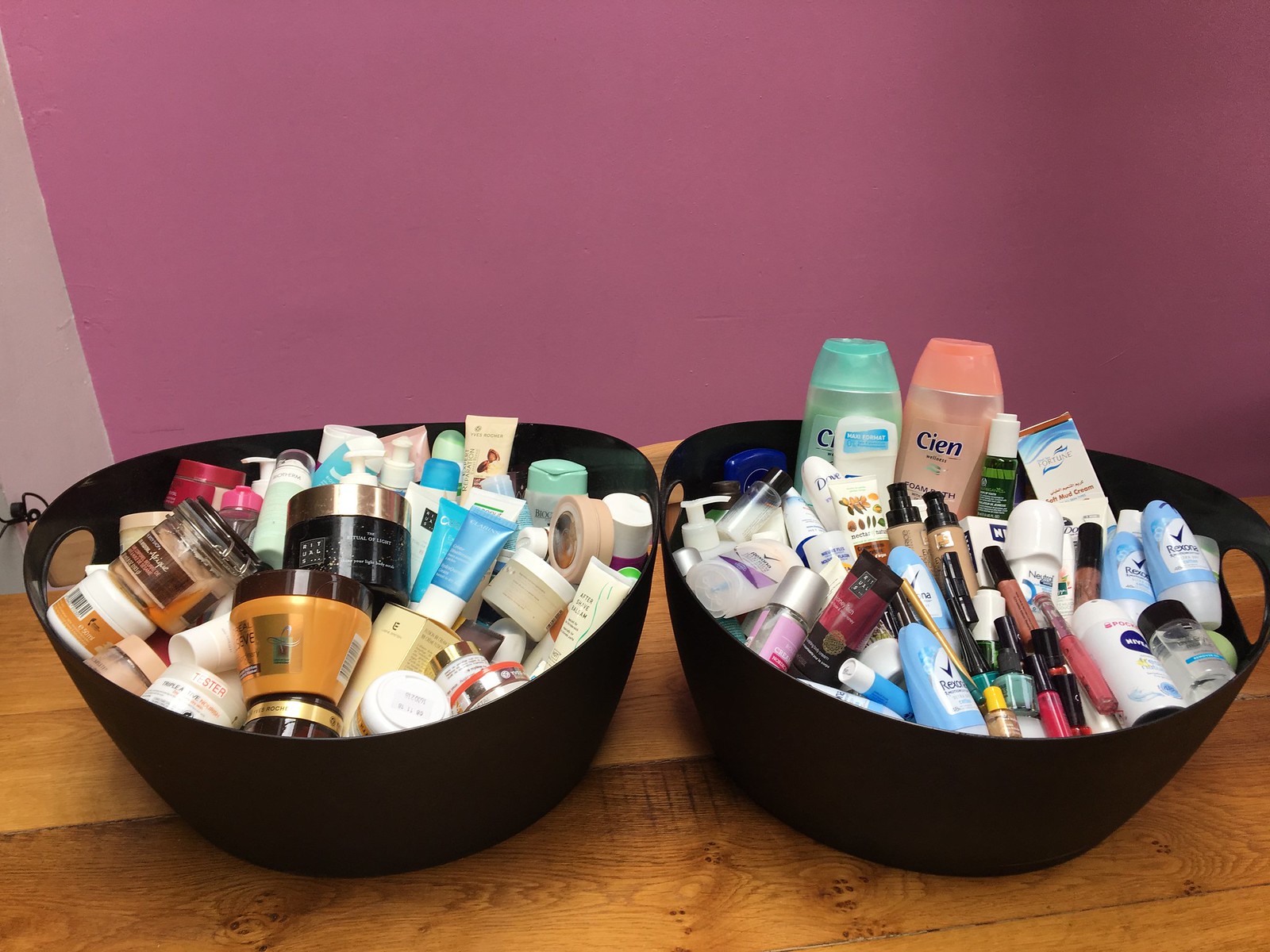In this vibrant color photograph, a striking purple backdrop dominates the scene, transitioning from a rich mauve hue on the right to a softer lilac shade on the left. The saturated colors create a vivid contrast with the foreground, where a wooden table is prominently placed. Atop the table, two large, low black plastic tote bins are crammed full of a myriad of skincare and beauty products. 

The bin on the left overflows with at least 30 different items, ranging from blue tubes, green flip-top bottles, orange jars, pink flip-top containers, to red jars—possibly Olay products—all of various brands and types. The bright, colorful packaging creates a lively patchwork within the bin. 

The bin on the right is similarly packed with an assortment of beauty products, including two tall bottles from the brand Cien, one green and one peachy colored, possibly shampoo and conditioner. Among these are makeup items such as foundation, lipstick, and eye pencils, alongside other personal care products like deodorant, evidenced by the familiar packaging with a check mark. Each bin showcases an eclectic collection, reflecting the variety and abundance of modern skincare and cosmetic products.